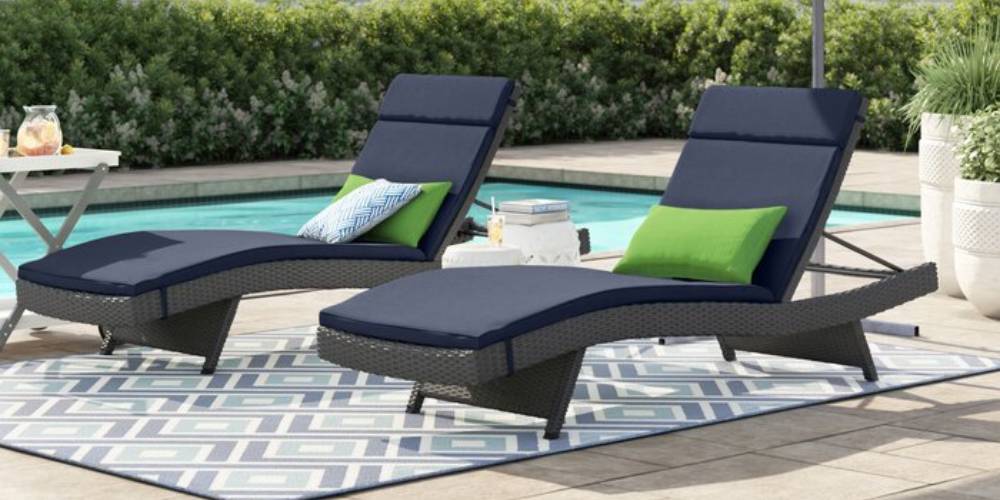The image depicts a serene and inviting outdoor setting, reminiscent of a high-end catalog. At the forefront are two comfortable, semi-reclined chaise lounges positioned on a blue and white diamond-patterned outdoor rug. Each lounge is adorned with pillows for added comfort—one chair featuring a solid green pillow alongside a patterned blue and white pillow, while the other supports a single green pillow. To the right of the leftmost chair stands a small side table bearing a pitcher of iced tea or another refreshing beverage.

In between the chairs is another small table, holding two books and an additional glass, suggesting a leisurely atmosphere perfect for reading and relaxation. The backdrop features a sparkling in-ground pool with lush green shrubs lining the perimeter, providing privacy and a touch of nature. Adding to the aesthetic, two tall outdoor vases filled with verdant plants complement the scene. The overall mood is one of tranquility and comfort, ideal for a quiet retreat or vacation setting, with every detail emphasizing relaxation and elegance.